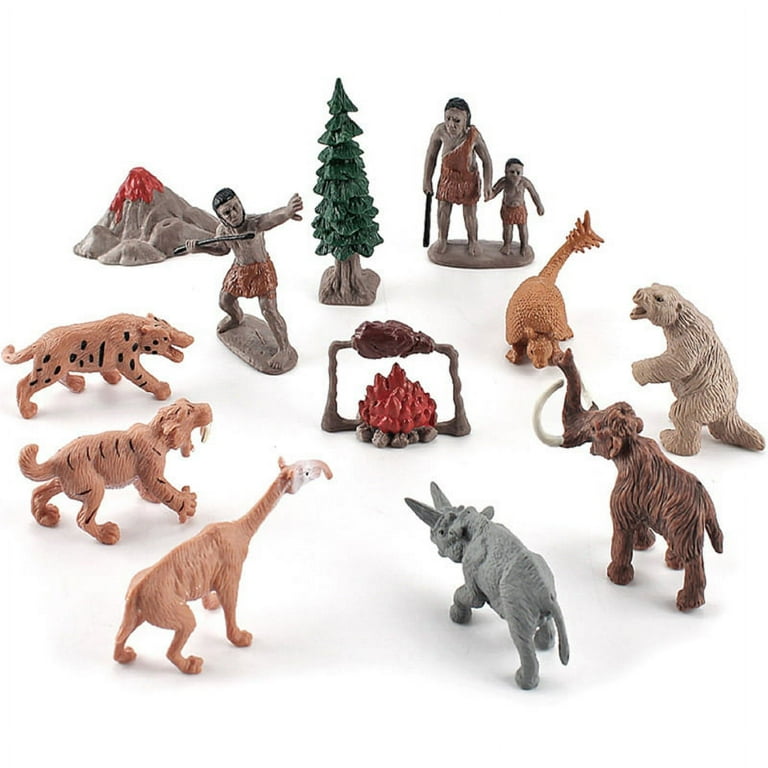Against a plain white background, a collection of roughly a dozen crude, minimally detailed figurines are displayed, likely designed for children. These small, predominantly green-painted plastic figures include a rudimentary depiction of a prehistoric scene. At the top, there's an evergreen tree and next to it, a small volcano with red lava dripping down its sides. The set includes various human figures: a bearded caveman in a red skirt wielding a spear, a cavewoman with a club, and a child holding her hand. Several animals resembling prehistoric ancestors are scattered around. There’s a brown woolly mammoth, a saber-toothed tiger, a gray rhinoceros, and a tan bear. Among them are also dinosaurs of various colors, including an orange one with a spiked tail, a tan one with a white head and curved snout, and a gray one with horns. Additional elements include a campfire with a piece of meat roasting on a spit and additional fauna that vaguely resemble a cheetah, a tiger, and a leopard. The overall craftsmanship is basic, featuring simple lines and a limited color palette.